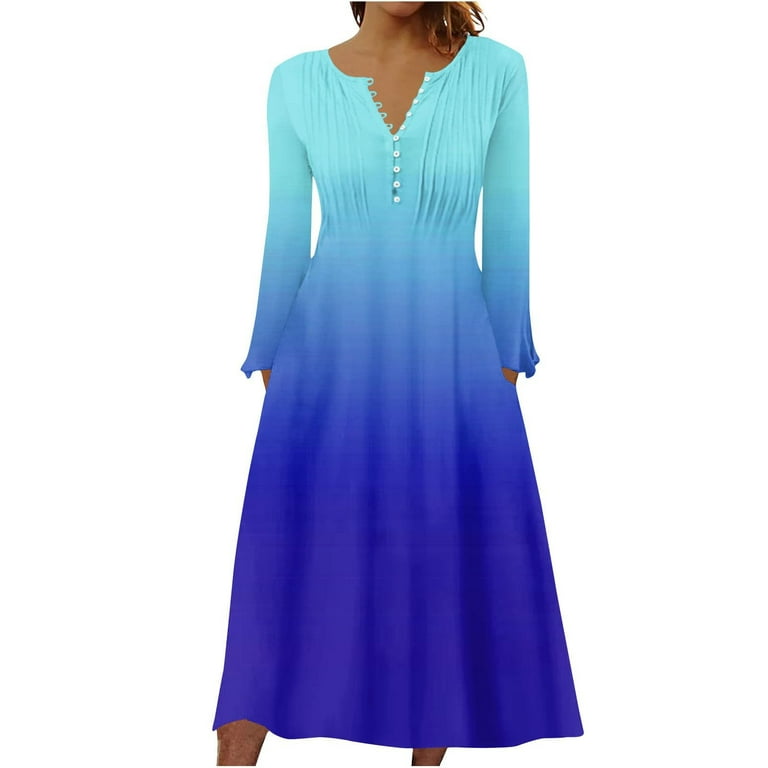This image appears to be a commercial product photo for a fashion catalog, showcasing a woman's dress. The model is shown from the chin down to just above the ankles, with only a hint of her brown hair visible near her neck. Emphasizing the dress, the photograph lacks a noticeable background, directing focus entirely on the garment.

The dress is characterized by a soft gradient that starts with a very light turquoise or teal at the top and transitions to a deep, ocean-like blue at the bottom. This gradient effect extends through the long sleeves as well, creating a harmonious color flow. The dress features a button-up front with about five of the white buttons undone to form a V-neckline, adding a touch of casual elegance. The chest area is detailed with ribbed vertical lines or pin tucks that extend down to an empire waist, where the gradient color becomes darker.

The sleeves are ruffled and flowy at the wrists, adding to the overall loose and flowing design of the dress. The dress has a very fluid and relaxed look, akin to linen, with a hemline that falls just above the ankles, making it versatile for various occasions. The model’s hands are tucked into pockets within the dress, further emphasizing the comfortable and effortless style of the garment.